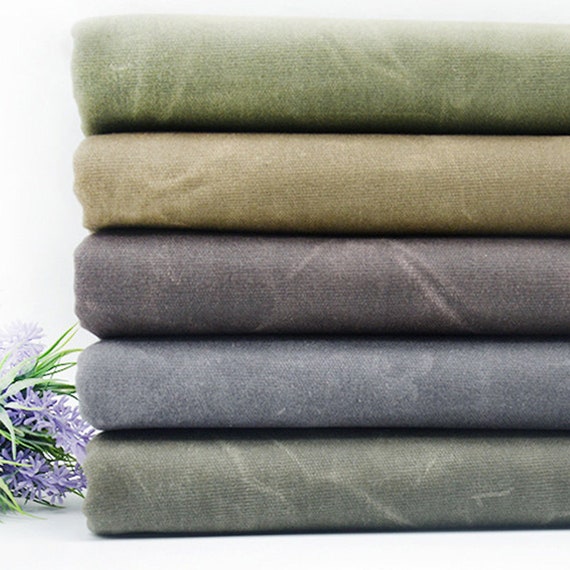This photograph features a neatly stacked pile of five folded fabrics, which could be blankets, towels, or sheets, arranged in descending order of size. The fabric at the top is a large, dark green piece, followed by a cream or tan-colored fabric that is slightly thinner. Below this is a medium-sized, dark purple fabric, and beneath that, a smaller blue one. At the bottom lies a grayish-green fabric, similar in size to the one in the middle. To the left of the stack, a sprig of blue flowers, possibly lilacs, is laid on its side. The background is a clean, white backdrop, giving the image a minimalist and organized appearance. The photograph is taken vertically, emphasizing the neatness and order of the stacked fabrics.